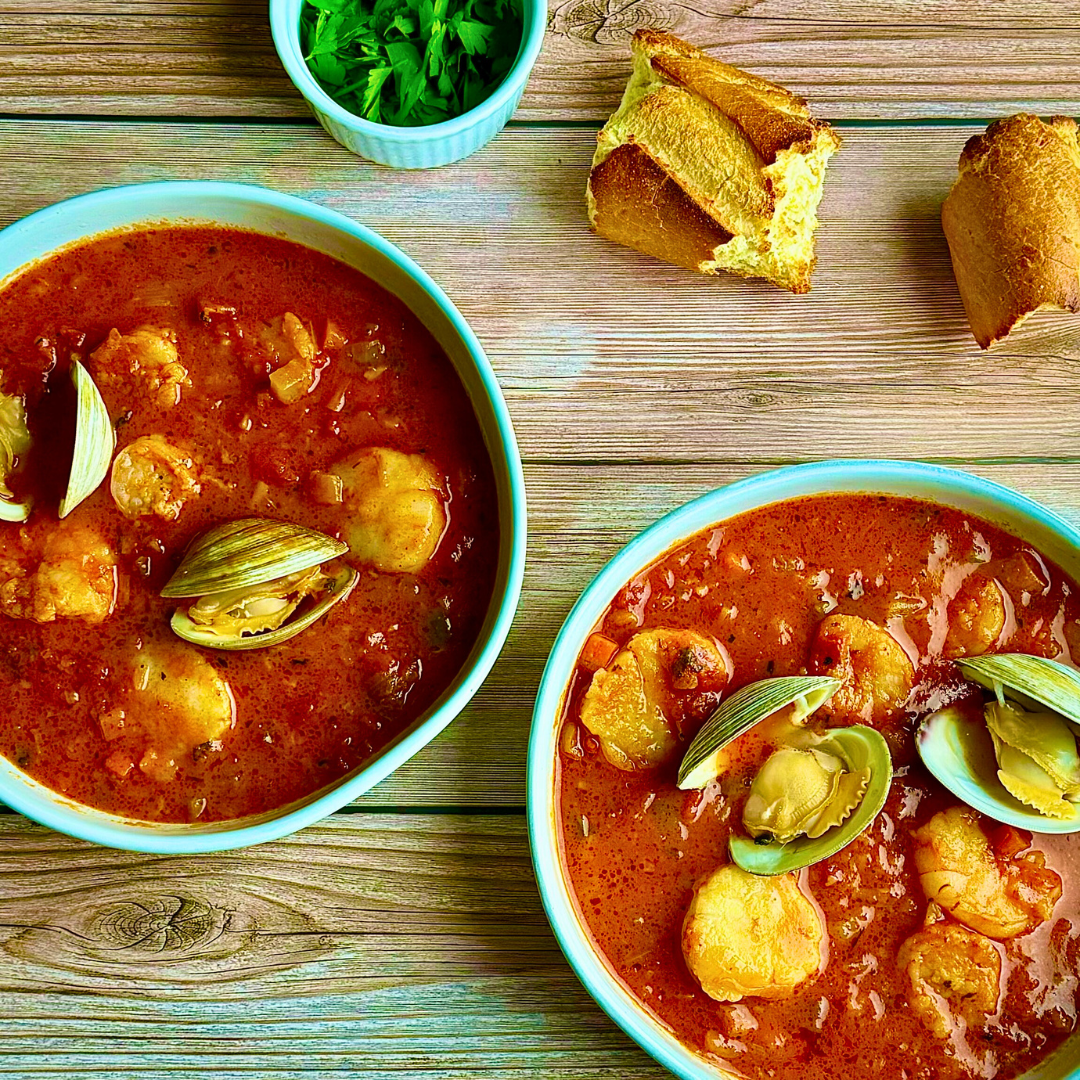This photograph showcases a rustic and inviting culinary scene on a medium-toned, light-colored wooden table with prominent wood grain and visible planks. At the center, two identical blue bowls brim with a rich, thick red soup, likely a tomato-based seafood stew. Within the soup, chunks of light-colored meat—possibly shrimp—and partway-open clams or oysters are visible, adding texture and flavor to the dish. Accompanying the bowls of soup are two pieces of crusty, rustic bread, perfect for sopping up the broth. To the left sits a small, white bowl with fluted sides, filled with chopped green herbs—likely cilantro or parsley—ready to garnish the dish. The overall presentation suggests a hearty, comforting meal with a touch of rustic charm.